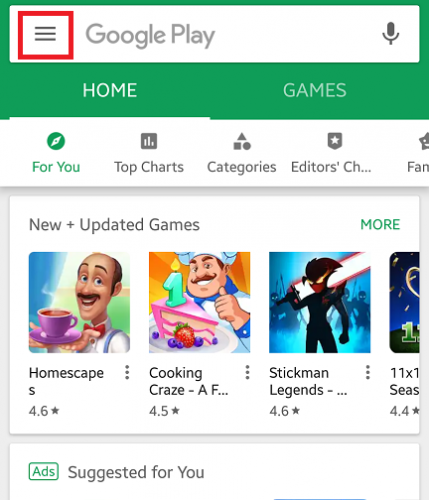This is a detailed screenshot of the Google Play Store interface, captured from a mobile device. At the top of the screen, there is an emerald green header featuring a central white search bar. On the upper left corner of the header, a red-outlined area encloses three horizontal black lines, indicating the menu icon. Adjacent to this icon, the text 'Google Play' is prominently displayed, while a gray microphone icon is situated on the far right of the header, suggesting voice search functionality.

Directly below the green header, there's a navigation bar with the labels 'Home' and 'Games' in white text. Beneath this, a row of tabs includes 'For You' (highlighted in green), 'Top Charts', 'Categories', and 'Editor's Choice' (all in gray), each accompanied by an icon above them.

Further down, a white rectangular section presents a section title 'New and Updated Games' in black text on the upper left, with a green 'More' link on the upper right. This section features three and a quarter mobile game icons, showcasing 'Homescape', 'Cooking Craze', 'Stickman Legends', and a partially visible game, likely titled 'Eleven Something'.

At the bottom of the screen, another white section contains a rectangular button with 'Ads' written in green on a white background, followed by 'Suggested for You' in gray text. This detailed layout provides a comprehensive view of the app store's interface and its features.